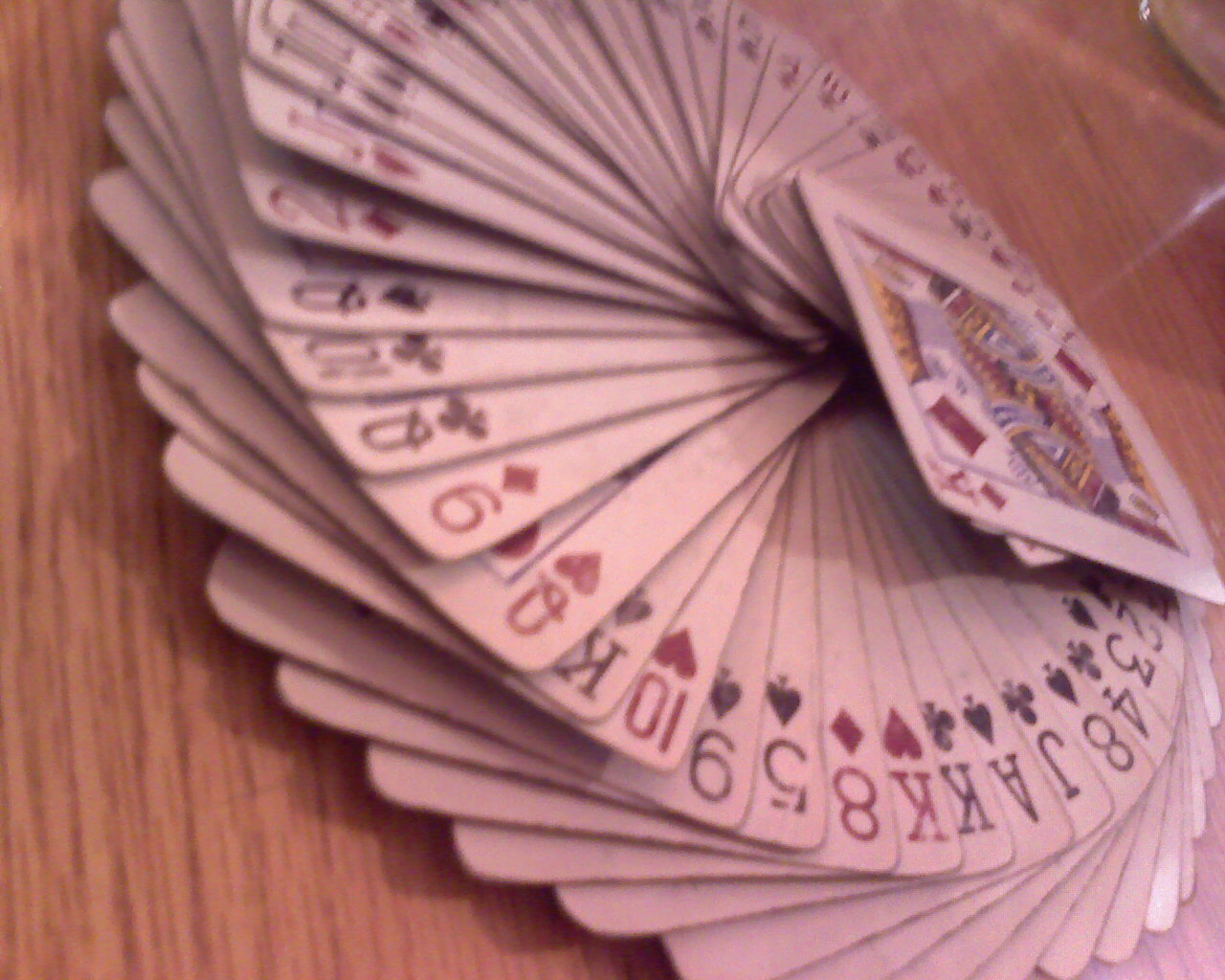The image features a wooden surface, possibly a table or floor, on which a deck of playing cards is arranged in a circular, spiral pattern. Shot from an angled top-side perspective, the photograph captures both the sides and the faces of the cards. These cards are the typical white-faced playing cards seen in standard decks. The most visible card is the King of Diamonds, placed prominently at the top. The cards are not in any specific sequential order but are spread out randomly in the spiral. Below the King of Diamonds, various cards are discernible, including the 2 and 3 of Spades, the 4 of Clubs, the 8 of Spades, the Jack of Clubs, the Ace of Spades, the King of Clubs, the King of Hearts, the 8 of Diamonds, the 5 and 9 of Spades, the 10 of Hearts, the King of Spades, the Queen of Hearts, the 9 of Diamonds, the Queen of Clubs, the 10 of Clubs, the Queen of Spades, and the 2 of Diamonds. The remaining cards blur into the background, making their identities hard to decipher.